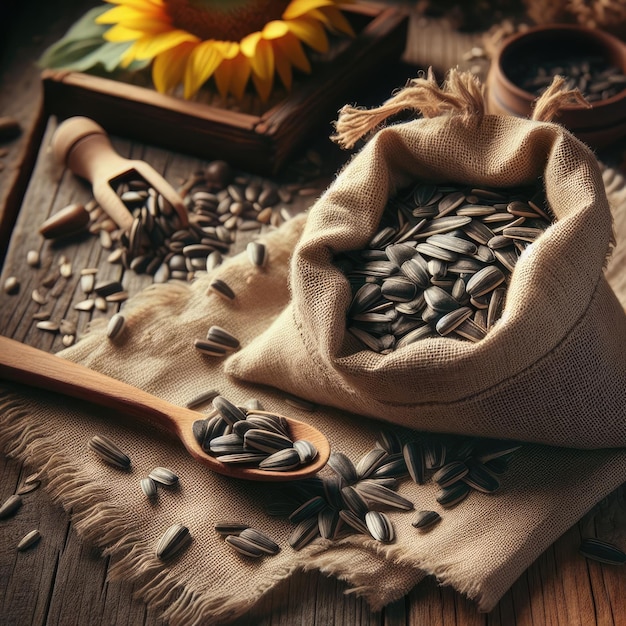A meticulously arranged still life photograph showcases a rustic yet refined table setting. A textured burlap fabric is elegantly draped across the wooden table, forming the backdrop for the scene. At the center, an open burlap sack is artfully displayed, its top folded down to reveal a bounty of sunflower seeds inside. A beautifully crafted wooden spoon, filled with sunflower seeds, lies in front of the sack, echoing its rustic charm. To the side, a wooden tray features a lifelike silk sunflower, adding a touch of vibrant color and thematic consistency. Scattered across the table are various tools, possibly nutcrackers, alongside a sprinkling of sunflower seeds, enhancing the organic and inviting atmosphere of the composition.